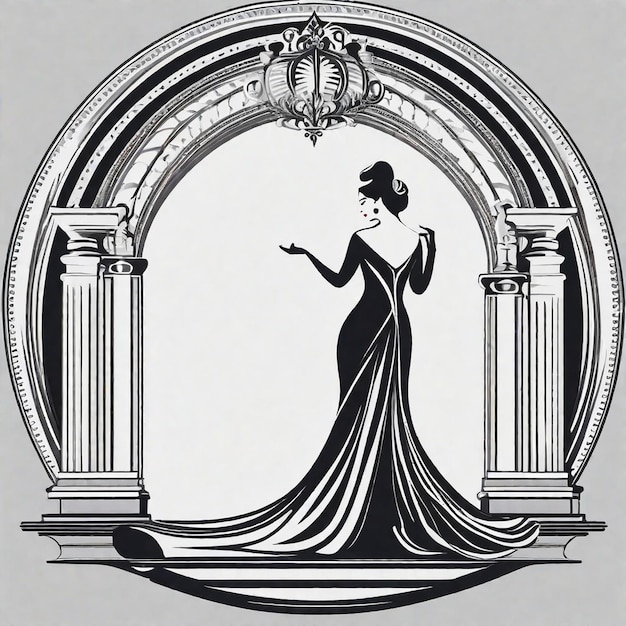This black and white drawing depicts a woman from the mid-20th century, probably the 1940s or 1950s, dressed in an elegant, floor-length black gown with a long train trailing about six feet behind her. The gown has long sleeves and black gloves, featuring a deep V-shaped back, revealing the midsection of her back. Her hair is styled in an intricate updo, resembling a duck on top of her head, and she wears black earrings. The woman stands on a step, striking a subtly elegant pose with her right hand extended while her left hand rests against her body. Two stone columns flank her on either side as she stands beneath a semi-circular entrance adorned with detailed engravings. The entire scene is rendered in shades of black, white, and gray, evoking a timeless, vintage atmosphere.